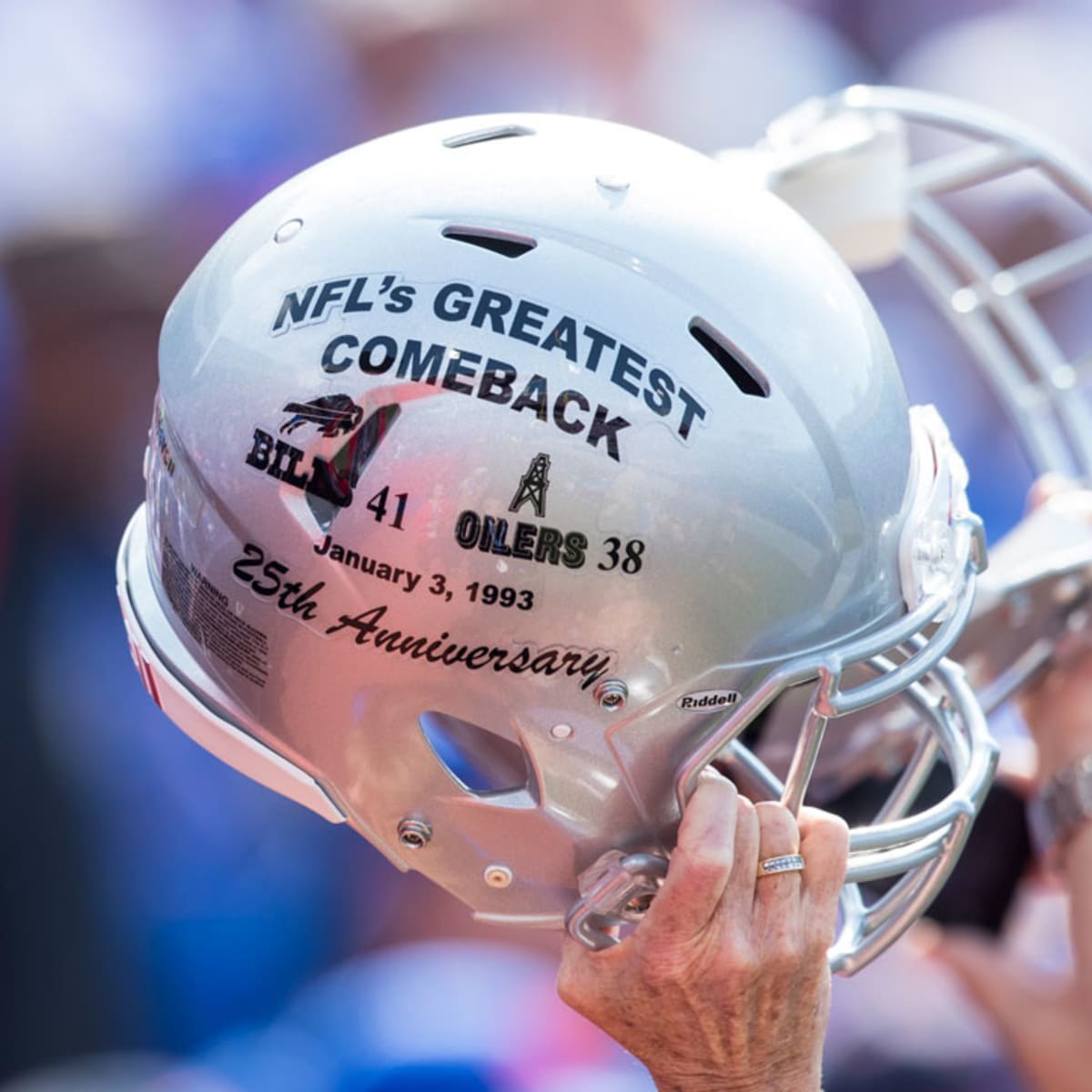The photograph showcases a silver Riddell football helmet, which is being held up by an older individual's hand adorned with sun spots and a diamond ring on the ring finger. The helmet prominently features black lettering that commemorates "NFL's Greatest Comeback," detailing the historic Bills versus Oilers game with a final score of 41-38 on January 3, 1993. The words "25th Anniversary" are written in a distinct script font. The helmet exhibits a full silver face guard, angled towards the right side of the image. The background is blurry, but it hints at a scene with individuals and blurred colors in hues of blue, white, and red, adding to the celebratory ambiance of the captured moment.